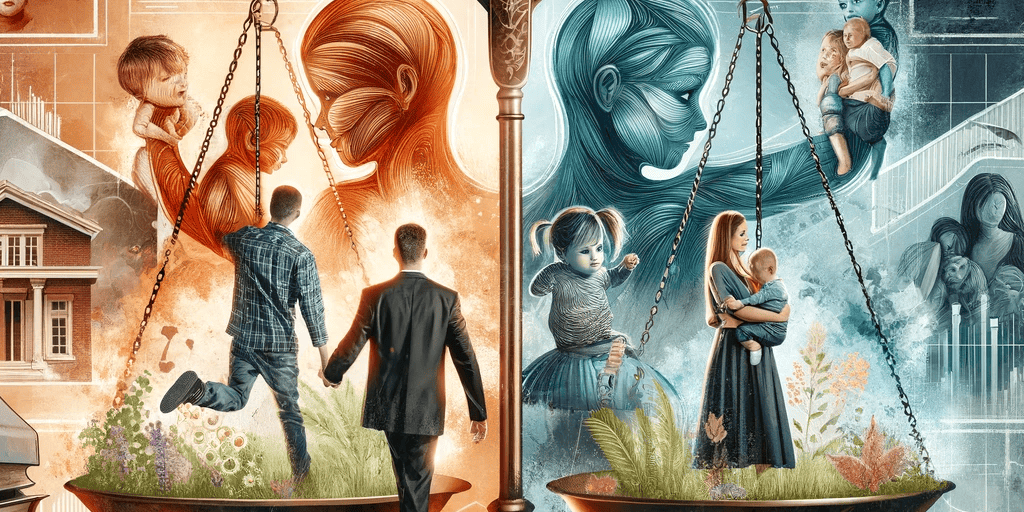The artwork portrays a poignant family scene split into two contrasting halves by an old-fashioned, golden copper set of scales, symbolizing a balance in family dynamics. The left side is bathed in warm, orange-golden hues, depicting two men walking away from the viewer; one in a blue plaid shirt and jeans, the other in a suit. They move towards the balancing bowl of the scale, which also holds additional abstract images of people and a house, suggesting the weight of responsibility and everyday life. The right side, dominated by serene light teal and blue tones, features a mother depicted in a muscled, almost skinless artistic style, standing with a young child in her arm and another on her shoulder, encased in greenery and flowers that add a softer element to the scene. These figures are mirrored by indistinct children in the backdrop, expressing subtle emotions that highlight the intrinsic juggling act of familial roles and burdens. The central golden pole of the scale acts as a stark division, accentuating the contrasting environments and the delicate equilibrium of family life.